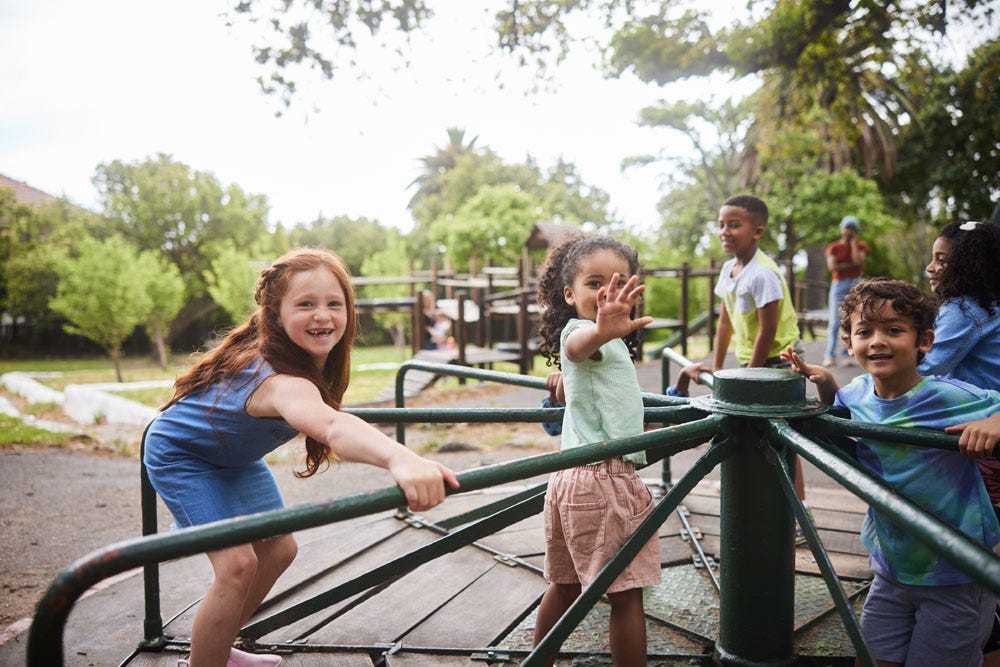In a bustling playground bathed in daylight, a bright white sky overhead, a group of children gleefully spin on a large circular piece of playground equipment resembling an old-fashioned merry-go-round. The surrounding scene is vibrant with an array of trees, both mature and recently planted, creating a lush backdrop. The focal point is the children, all smiling broadly and standing on a wooden platform as they hold onto the railings. 

On the left edge of the wheel, a little Caucasian girl around seven years old with long red hair, dressed in a blue jumpsuit, stands poised and animated. Towards the center, slightly to the right, stands an African-American girl, approximately five years old, her shoulder-length curly hair bouncing as she raises a hand. She wears a green top paired with orange shorts. Next to her is an African-American boy, around six or seven, wearing a yellow t-shirt and shorts. Beside him stands a young Hispanic boy, about the same age, donning a blue t-shirt and matching shorts with curly hair.

Behind them, partially obscured, is another African-American girl, about the same age, dressed in a long-sleeved blue shirt. All the children appear joyful and engaged in the spinning activity. In the background, amidst additional play structures, an adult is seen, possibly taking a photograph, adding a touch of supervision and care to the lively scene.